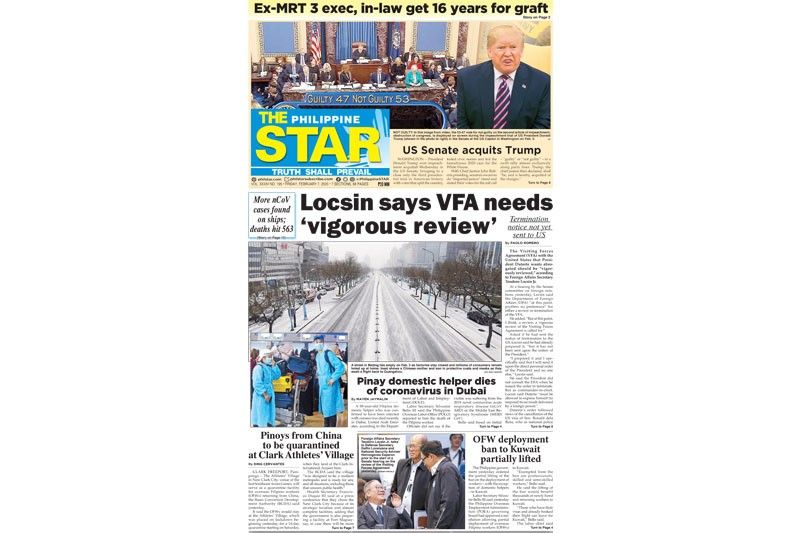Front Page of "The Philippine Star":

[Header]
- **The Philippine Star**: The top left section of the front page prominently features "The Philippine Star" logo. The word "The" and "Star" are in yellow font, and "Philippine" is in white font, all set against a blue background. Beneath the logo, in smaller white text, the slogan "Truth Shall Prevail" is displayed.

[Main Article and Image]
- **U.S. Senate Acquits Trump**: The main section presents an image showcasing a political assembly with board members, including the U.S. flag and another flag which may be that of the Philippines. Featured on the right side of the image is former U.S. President Donald Trump, with a caption detailing the impeachment trial results: "Guilty: 47, Not Guilty: 53."

[Additional Articles]
1. **Ex-MRT3 Exec and In-Law Sentenced**: Above the main picture, a headline reads, "EX-MRT3 EXEC, IN-LAW GETS 16 YEARS FOR GRAFT."
2. **Call for VFA Review**: At the center of the page, an article headlined "Loc-sin Says VFA Needs Vigorous Review" is framed against a white background.
3. **Termination Notice Not Sent to U.S.**: To the right of the main image, another article discusses the suspension, headlined "Termination Notice Not Sent to U.S."

[Sub-Articles]
- **Snowy City Image**: Displays a picture of a city with snowy roads, aligning with an article about cold weather conditions.
- **Coronavirus-related News**: 
  - "PNA Domestic Helper Dies of Coronavirus in Dubai": A tragic account of a Filipino domestic worker succumbing to the virus, accompanied by an image of people in masks and medical gowns.
  - "Panois from China to be Quarantined at Clark's Athletic Village": Describes quarantine measures for Filipinos returning from China.
  - "OFW Deployment Ban to Kuwait Partially Lifted": Reporting on the partial lifting of the Overseas Filipino Workers deployment ban to Kuwait.

By delivering thorough and vivid details, this formatted caption offers readers a comprehensive glance at the newspaper's front page.